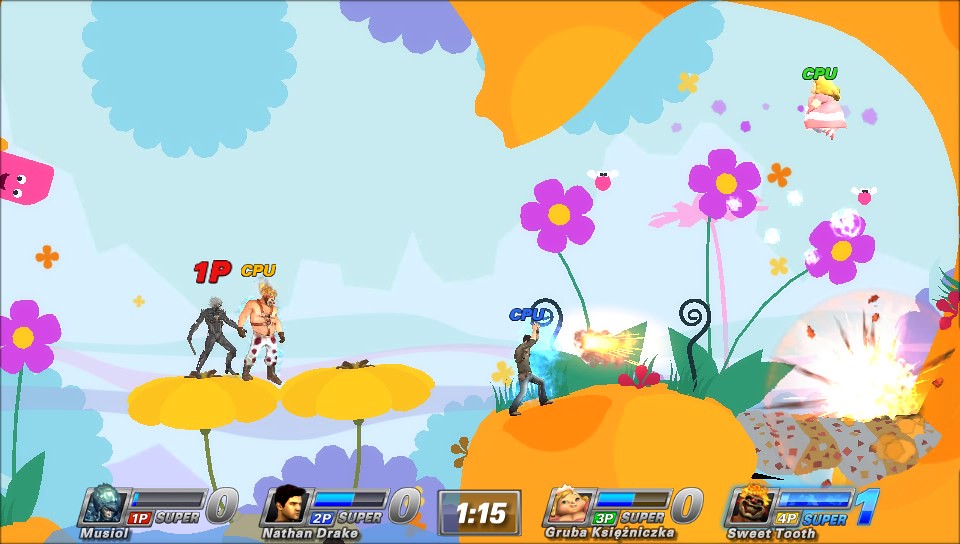This image appears to be a screenshot from a video game. Along the bottom of the screen, there are four character profiles: "Musiel," "Nathan Drake," "Gruba" (with an unpronounceable suffix), and "Sweet Tooth." Each character has a corresponding progress bar filled with a blue line, indicating a certain status—possibly health, magic, or experience. Musiel's bar is nearly empty, while Sweet Tooth's bar is completely filled. Nathan Drake and the third character (Gruba) also have almost empty bars. Additionally, Musiel, Nathan Drake, and Gruba have a numerical value of zero next to their bars, whereas Sweet Tooth has a value of one.

The background features a vivid, cartoon-like environment with numerous flowers and characters standing atop them. The scene is bright and colorful, dotted with orange elements and curved structures, creating an engaging and whimsical visual experience.